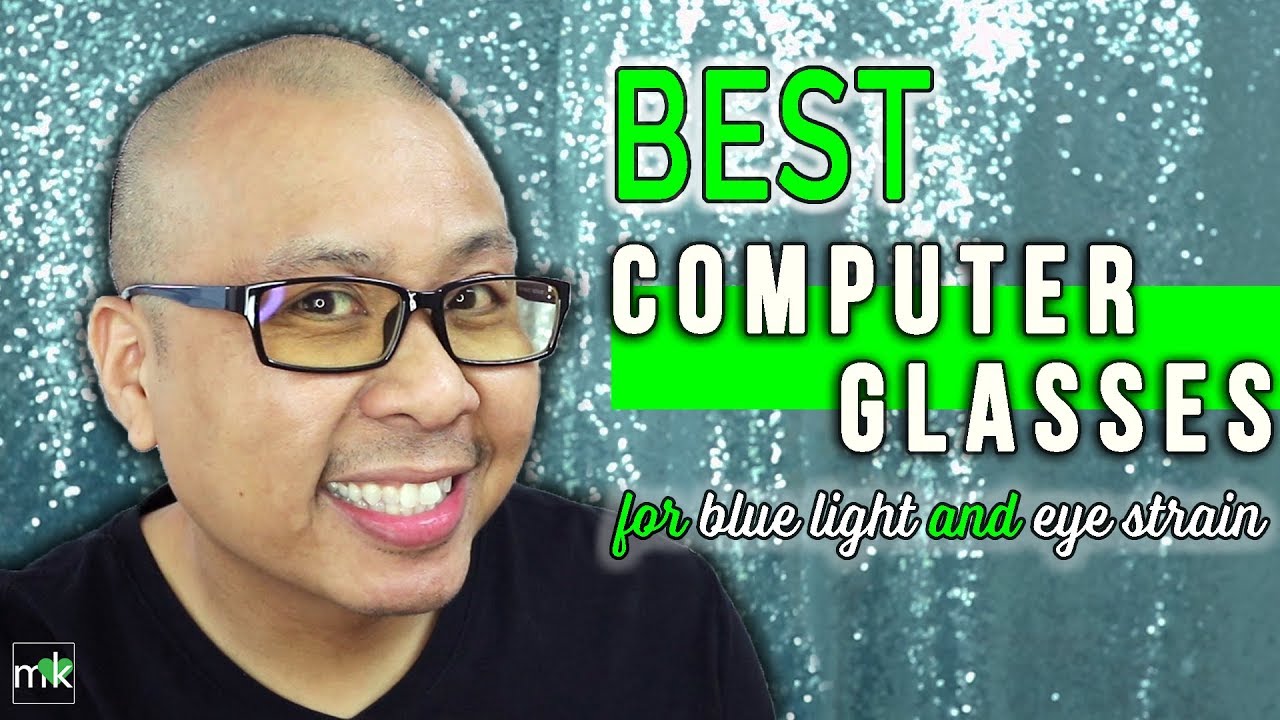The image is an advertisement for computer glasses designed to reduce blue light and eye strain. On the left side, a man, possibly Hispanic or Asian with a low-cut hairstyle, sports a black shirt and black-rimmed glasses, flashing a broad smile. The background behind him features a shiny, sequined fabric in a light, seafoam green color. In the bottom left corner, there is a logo featuring a white square with the letters "MK" and a green heart superimposed over the "K." On the right side of the image, bold green text proclaims "BEST," followed by "computer glasses" in white text on a green band. Below this, the phrase reads "for blue light and eye strain" in alternating green and white text.